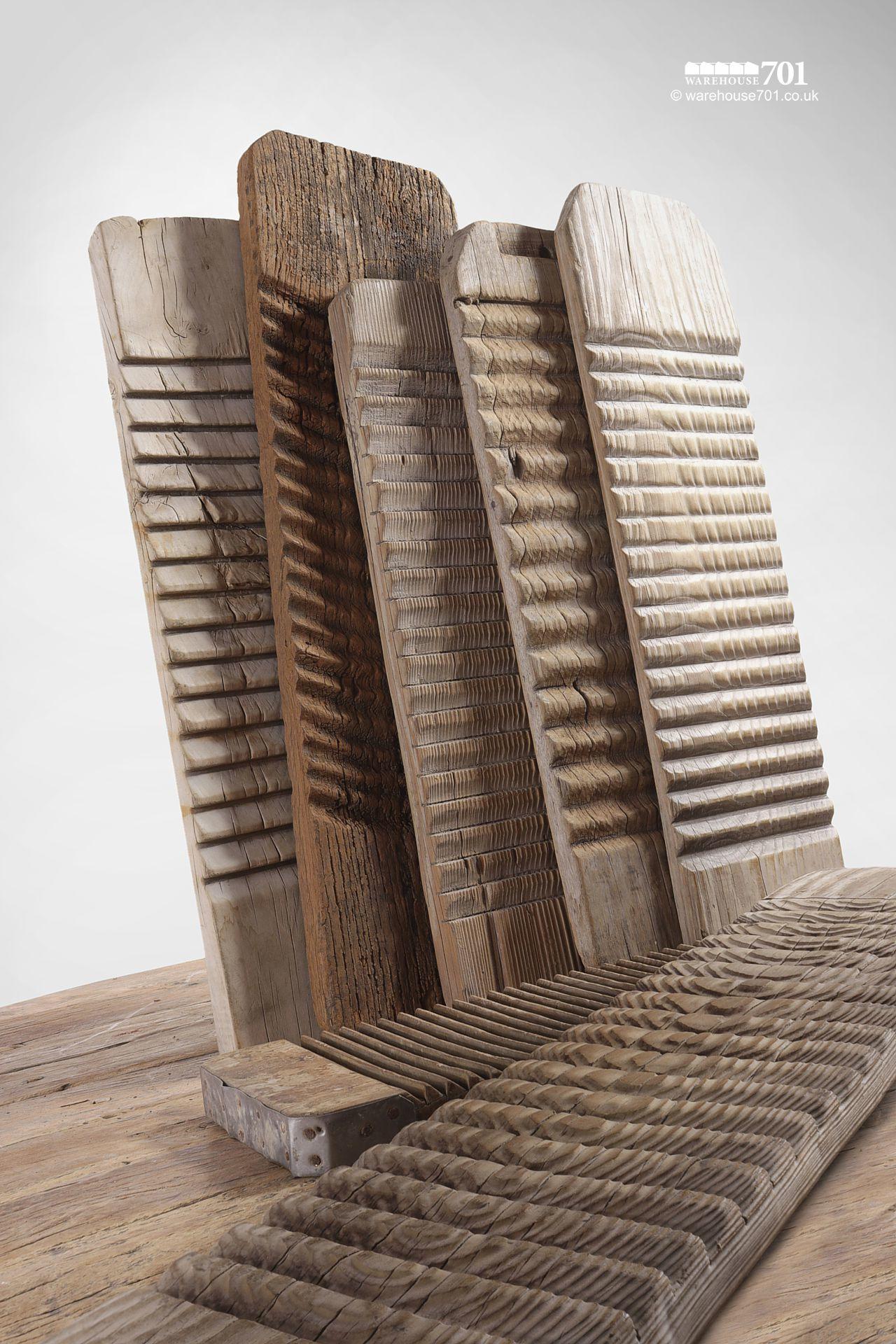The photograph depicts a collection of antique wooden washboards lying and leaning on a wooden floor against a grayish-white backdrop. Among the variety, there are at least five prominently standing upright. These washboards come in different tones of wood, with one being dark brown and others a light whitish-brown. They display distinct wood grain patterns and have grooves or ridged surfaces running through their centers. Some appear narrower and more uniformly ridged, resembling the texture of washboards traditionally used for washing clothes. Others have rounded ridges, similar to the undulating mounds found in skiing moguls. Additionally, two unfinished, unstained boards lie on the bottom right portion of the image, further contributing to the rustic and antique aesthetic of the scene. The arrangement and varied textures highlight their historical usage and craftsmanship.